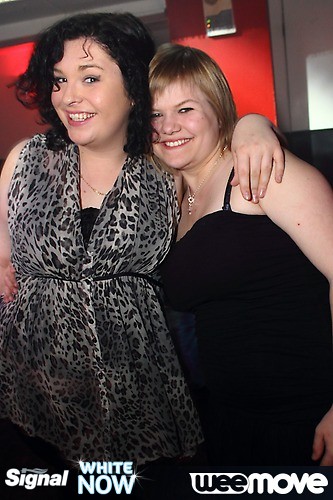The image captures two smiling women embracing each other against a predominantly red background, indicative of a celebratory or event setting. Both appear to be in their 30s and are of Caucasian descent. The woman on the left, with short curly black hair, is wearing a gray leopard print dress and has her left arm around the woman on the right, who has short thin blonde hair and is dressed in a black strappy dress. Both women are also adorned with necklaces. The background features a red wall, and the bottom of the image contains promotional text and logos in white and light blue fonts, reading "Signal," "White Now," and "We Move" (with "We" stylized as "W-E-E").